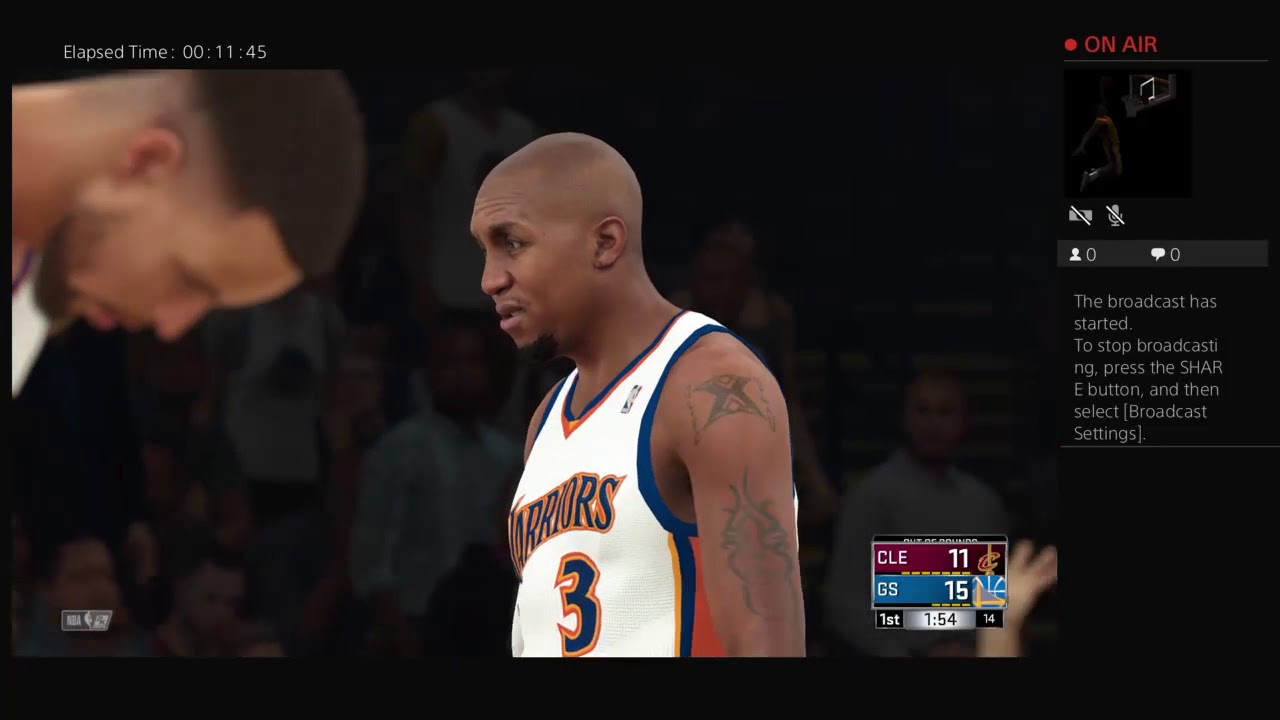The image appears to be a screenshot from a computer-animated video game featuring a basketball match. The game's graphics display detailed representations of basketball players on the court, with a computer-generated audience visible in the stands behind them, adding to the immersive atmosphere. 

On the far right of the screen, there's an "On Air" indicator, suggesting that the game is being live-streamed. Beneath this indicator, there is a notification stating, "The broadcast has started. To stop broadcasting, press the share button and then select broadcast settings," indicating that the streaming session is active and providing instructions on how to end it.

At the bottom of the screen, a score bar is visible, showing the current score as CLE 11 (presumably Cleveland) and GS 15 (presumably Golden State). The timer indicates that there are 1 minute and 54 seconds remaining in the first quarter, providing context for the stage of the game.